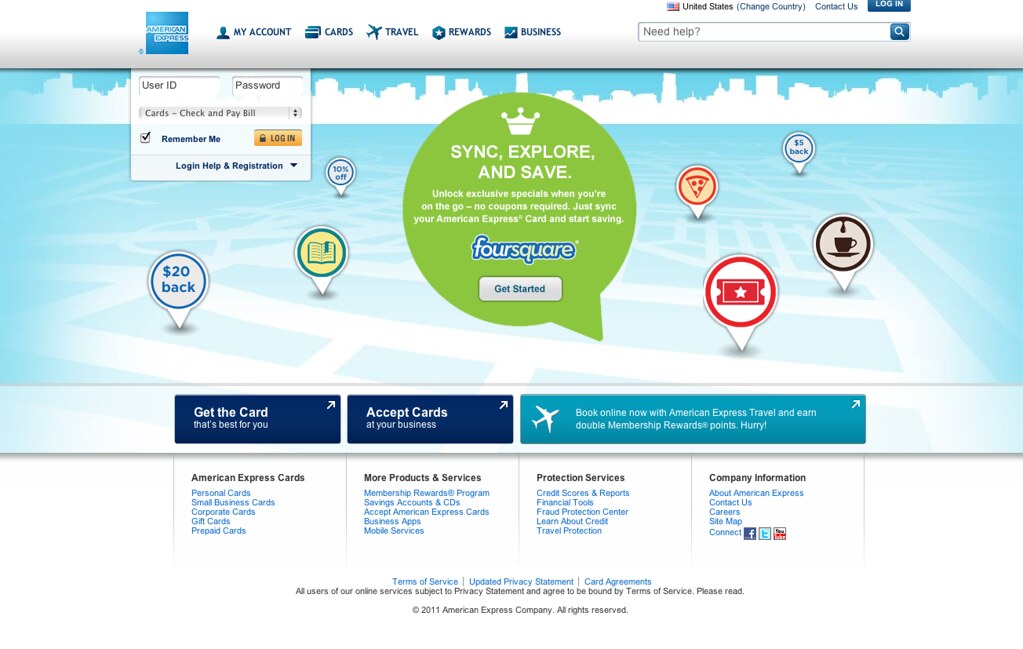**Caption:**
This detailed image showcases the homepage of the American Express website, identifiable by the URL "americanexpress.com." The top navigation bar prominently features tabs such as "My Account," "Cards," "Travel," "Rewards," and "Business," all accented in a sleek blue font accompanied by matching blue icons. On the top-right corner, a user-friendly search bar presents the prompt "Need Help?" alongside other options including "United States," "Change Country," "Contact Us," and a blue "Login" button.

Centrally, a standout green speech bubble with white text encourages users to "Sync, Explore and Save," highlighting the benefit of unlocking exclusive offers without the need for coupons. Users are instructed to sync their American Express card with the FourSquare app to start saving. Accompanying this call-to-action, several icons such as pizza, coffee, coupon, books, cashback, and a 10% off indicator enrich the visual appeal. The cashback amount displayed is $20. Below this, a prominent "Get Started" button invites user engagement.

The top-right quadrant of this section contains a sign-in bar prompting users for their "User ID," "Password," "Card Check," and "PayPal" information, complete with a yellow "Login" button and additional options like "Remember Me," "Login Help," and "Register" links. This section is set against a blue and white background for readability.

Towards the bottom of the page, additional tabs guide users to explore more features: "Get the Card that's Best for You," "Accept the Card at Your Business," "Book Online Now with American Express Travel," and "Enterprise Membership Rewards Points." The overall design is clean, intuitive, and aims to provide a seamless user experience.